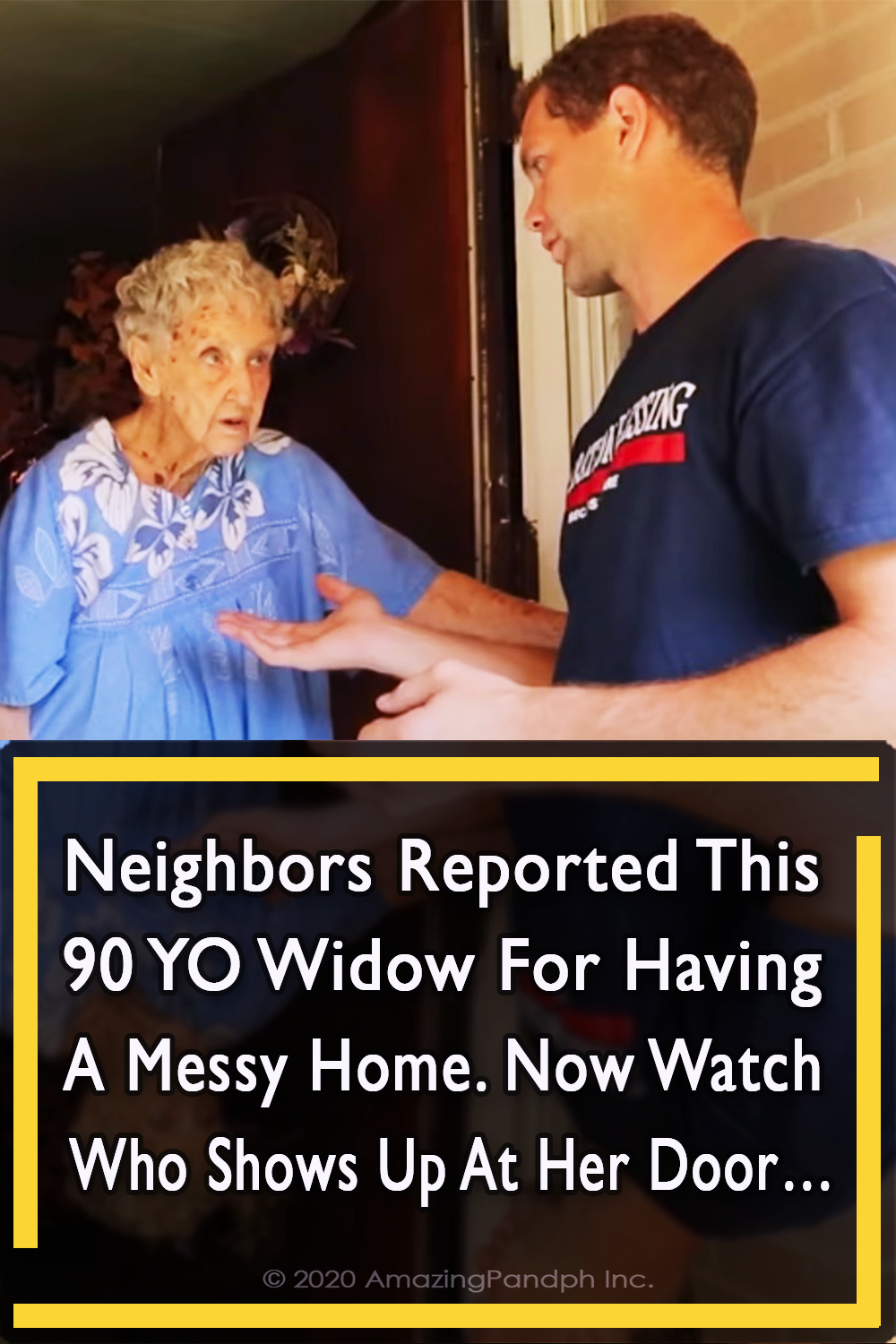The image depicts a vertical rectangular scene focusing on an interaction between an elderly woman and a younger man at her front door. The elderly woman, appearing to be around 90 years old, has short white hair and is wearing a blue floral nightgown. She looks somewhat confused as she holds the wooden door, framed in white, open. The younger man, dressed in a dark blue t-shirt with partly obscured white writing, extends his hand towards her as if explaining something. To the right of the door is a red brick wall with white mortar. The lower part of the image features a black box outlined in a yellow frame, containing white text that reads, "Neighbors reported this 90-year-old widow for having a messy home. Now watch who shows up at her door...". The image is copyrighted 2020 by Amazing Pan DPH Incorporated.